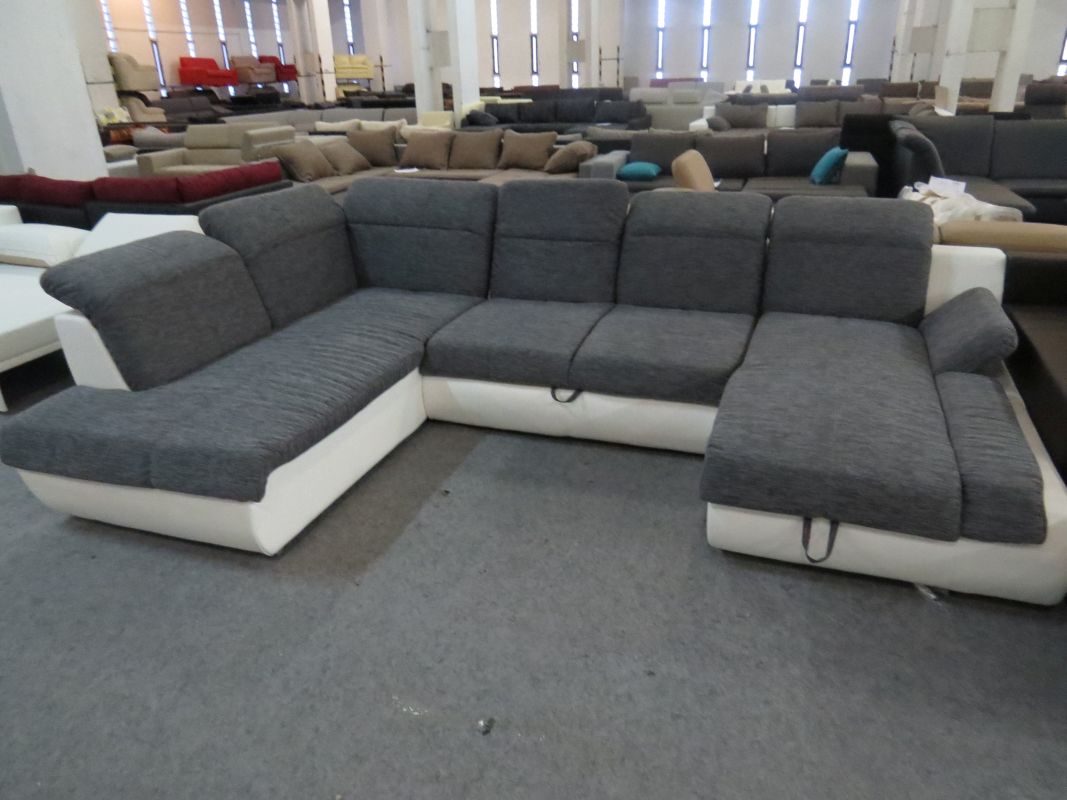The image captures the interior of a spacious furniture store featuring a wide variety of seating options. The focal point in the foreground is a modern, U-shaped sectional couch with a white base and dark linen gray cushions. The couch is detailed with sewn-in handles, suggesting hidden storage or adjustable features. Surrounding this central piece are numerous other couches in diverse colors, including blacks, whites, browns, reds, and greens, with varied designs and upholstery. In the background to the left, there's a multi-tiered shelf displaying large, loungy chairs. The store's ambiance is enhanced by unique windows in the back, which feature slender slits between columns that allow light to filter through, creating an interesting architectural effect. The floor is a sleek gray concrete, adding to the contemporary feel of the space. Visible columns also add structural elements to the open, airy layout of the store.